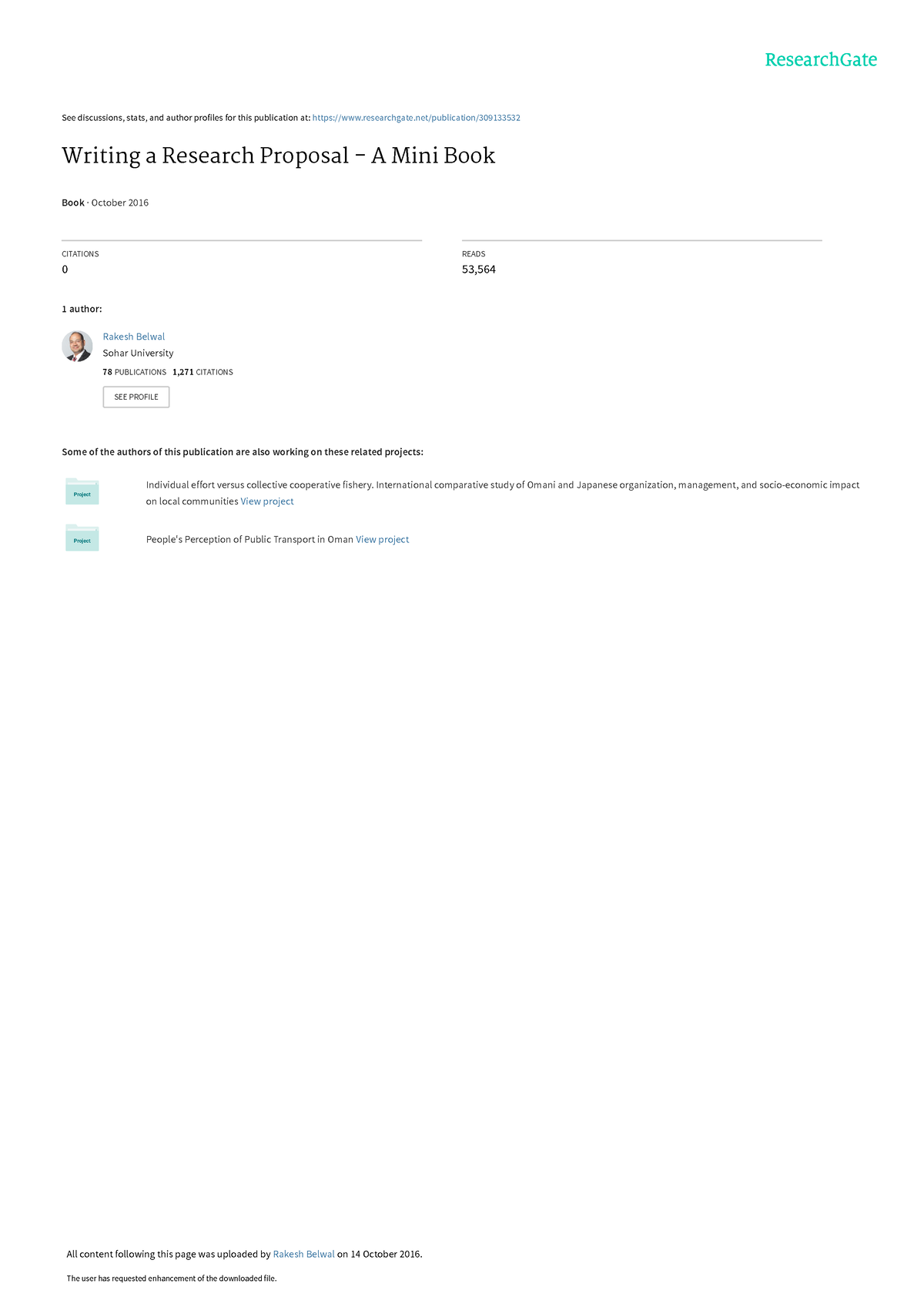The image is a screenshot of a section from a guide-like website, specifically a page on "ResearchGate." The top-right corner, highlighted in mint green, prominently displays "ResearchGate." On the top-left corner, the section title reads "Writing a Research Proposal: A Mini Book." Just below this title, the text indicates that this is a book published in October 2016. Further down, there is a citation count listed as "Zero" and, on the far right, a read count displaying "53,564." The left side of the screenshot also notes that there is "One Author," though the author's name is blurry and difficult to discern, possibly identifying a male author.